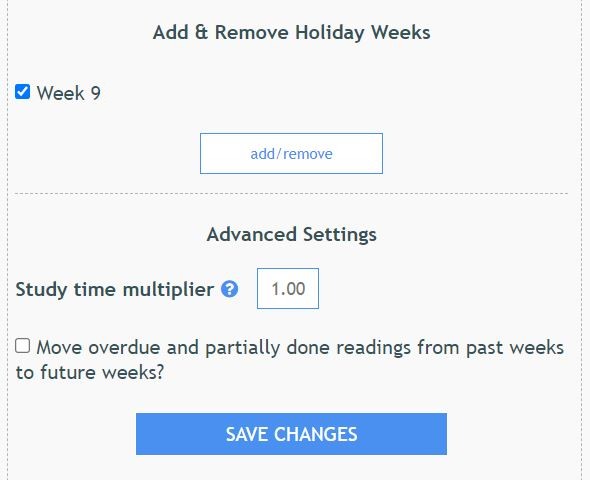A screenshot of a digital interface is presented. At the top of the interface, a section titled "Add and Remove Holodeck" is visible. Below this title is a blue box with a text entry field and a checkmark option that labels it "Add/Remove."

On the left column of the interface, a series of items is listed, including:

1. "Advanced Settings" - Indicated by dash marks.
2. "Study Time Multiplier" - This likely adjusts the intensity or duration of study time.
3. An icon of a circle with a question mark inside it, usually intended for help or additional information.

There is also a square option box indicating "1.0" which relates to the "Study Time Multiplier."

Inside this box, there's another checkbox labeled "Remove Overdub, Partially Done Readings from Past Weeks," which is unchecked. Additional prompts read "Two for Two Weeks" and mention "Concentration."

The background of the interface is grey, which seems to be the standard color for the page. The text is mostly grey, appearing grainy and of low quality. There are also dotted vertical lines visible, whose purpose is unclear in the image.